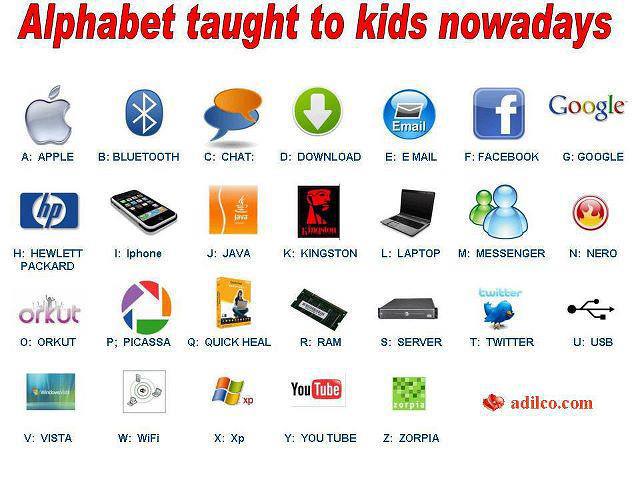This is a full-color, computer-generated image with no background, just a flat white canvas filled with rows of company and product logos designed to teach the alphabet. At the very top in bold red text, it reads "Alphabet Taught to Kids Nowadays." The image features each letter of the alphabet paired with a corresponding corporate or product logo, creating a modern-day educational chart. For example, 'A' showcases the Apple logo, 'B' displays the Bluetooth symbol, 'C' features a chat logo, 'F' has the Facebook logo, and 'Y' shows the YouTube logo. The logos appear slightly dated, representing designs from five to ten years ago. The alphabet grid is clearly organized into four rows, extending from 'A' to 'Z,' with notable entries like 'H' for Hewlett Packard, 'I' for iPhone, 'S' for server, and 'L' for laptop. At the bottom of the image, after the letter 'Z,' a small red text mentions "adlico.com."